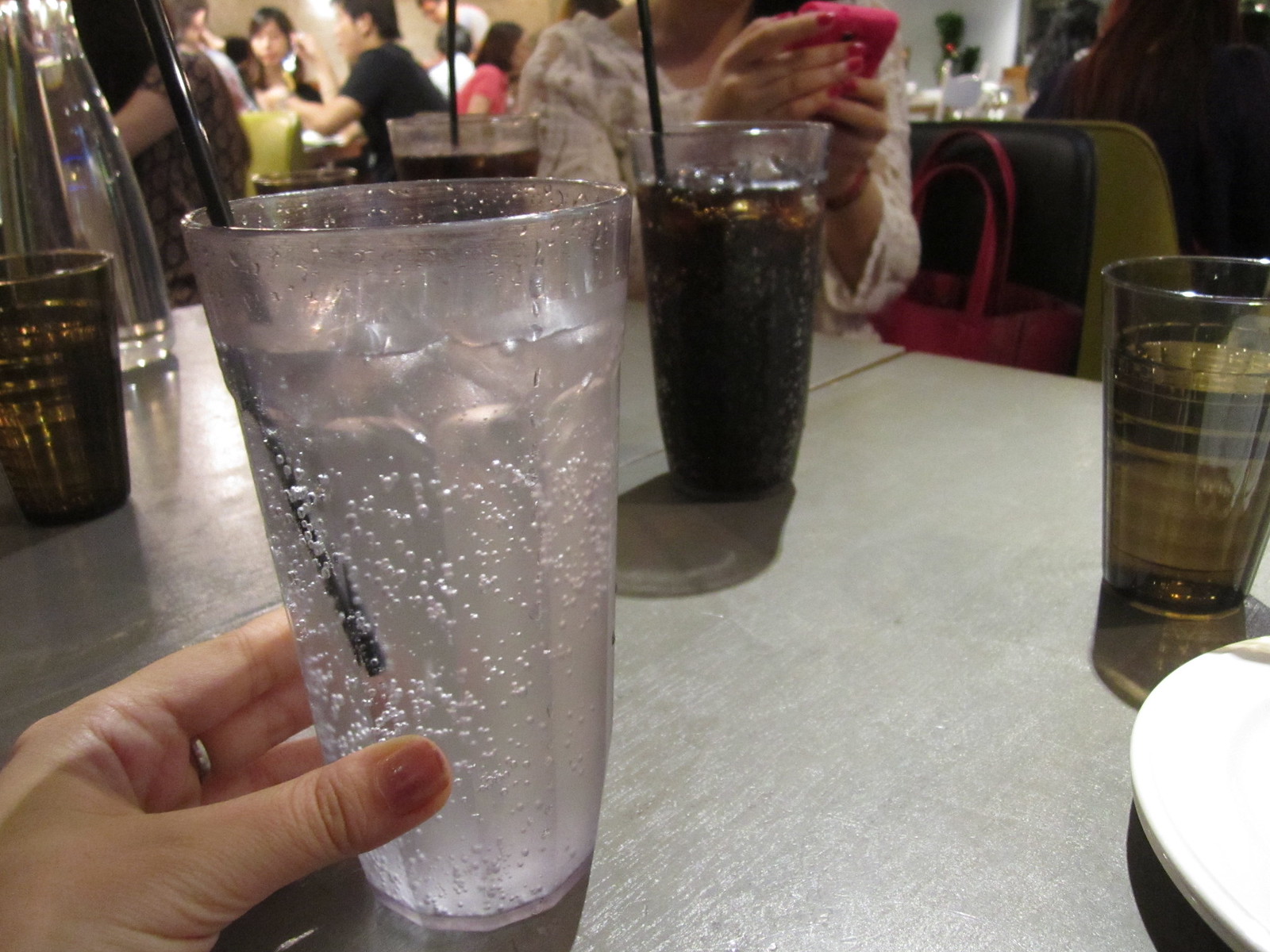In this color photograph taken inside a restaurant, the foreground captures a detailed scene of a tabletop with a glossy surface. A woman’s left hand, adorned with short nails polished in a rose pink hue, is holding a tall glass tumbler filled with a clear, bubbly liquid, likely Sprite, through which a black drinking straw protrudes. To the right of this glass, there is another identical glass filled with a dark brown, carbonated beverage, possibly Coca-Cola, also featuring a black straw. Opposite the woman, her friend is visible from the neck down, engrossed in her red cell phone, which she holds with both hands that are similarly polished with red nail polish. In the background, towards the top left of the image, a group of young Asian people, possibly a family, can be seen sitting around a table, engaged in their meals. Additional glasses, shorter with a smoked brown appearance and striped designs, are scattered on the table, contributing to the restaurant ambiance enhanced by the lighting that casts shadows of the drinks toward the foreground.